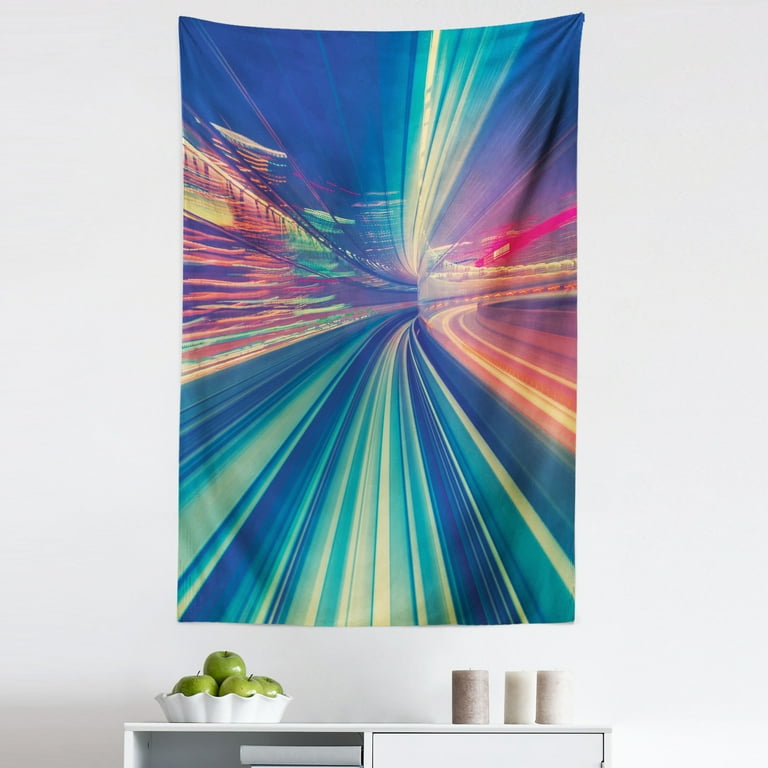This photograph features a minimalist home setting with a distinctively vibrant aesthetic. Central to the image is a white wall adorned with a vertically hanging, colorful fabric mural. The mural captures an abstract action shot, giving the impression of speeding through time or space with streaks of red, blue, yellow, and other vibrant colors emanating like bursts of light in all directions. Beneath this dynamic artwork sits a pristine white bookshelf. On the left side of the top surface of the bookshelf, a white, curly-lipped bowl houses four shiny green apples. On the right side, three light grey or beige candles are arranged in a somewhat haphazard fashion. The composition of the photograph blends a serene, minimalist ambiance with an energetic splash of color, creating a striking visual contrast.